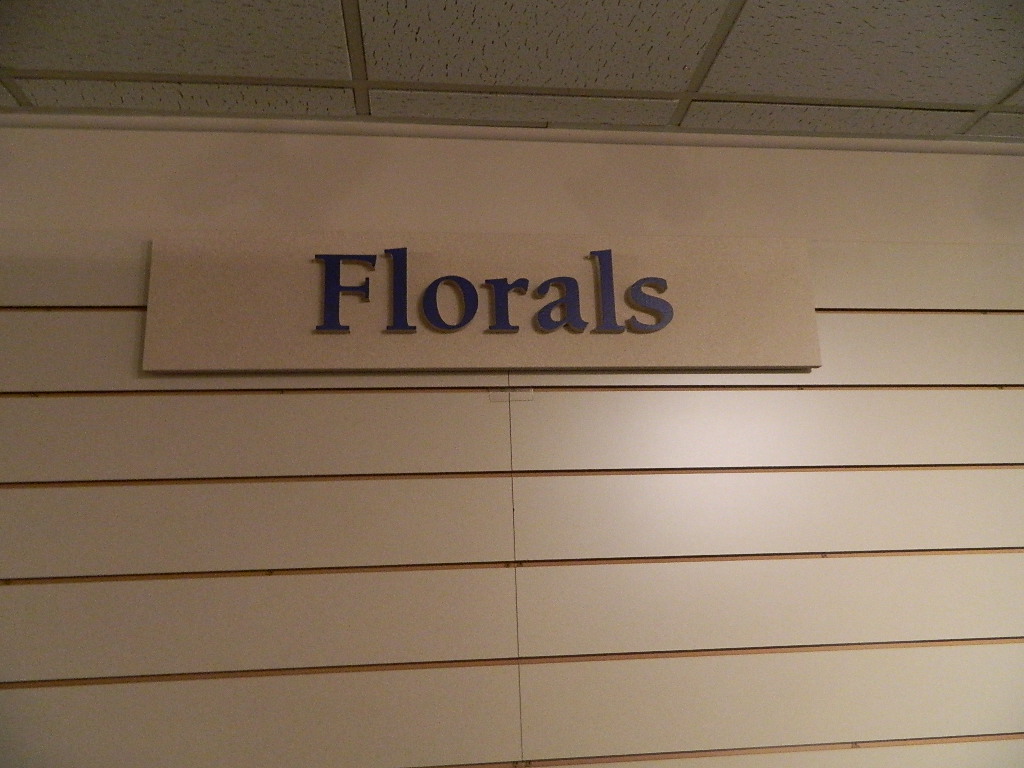This photograph captures the interior of a store, showcasing a section of a faux wall designed for display purposes. The wall, characterized by evenly spaced horizontal grooves, is intended for hanging various items. Positioned prominently at the center of the wall is a sign that reads "Florals" in black lettering. Above this arrangement, the ceiling features a typical grid pattern made of metal, accommodating recessed foam panels that rest within the wire framework. The wall extends seamlessly from the left to the right edge of the image, highlighting its uninterrupted span across the store's interior.